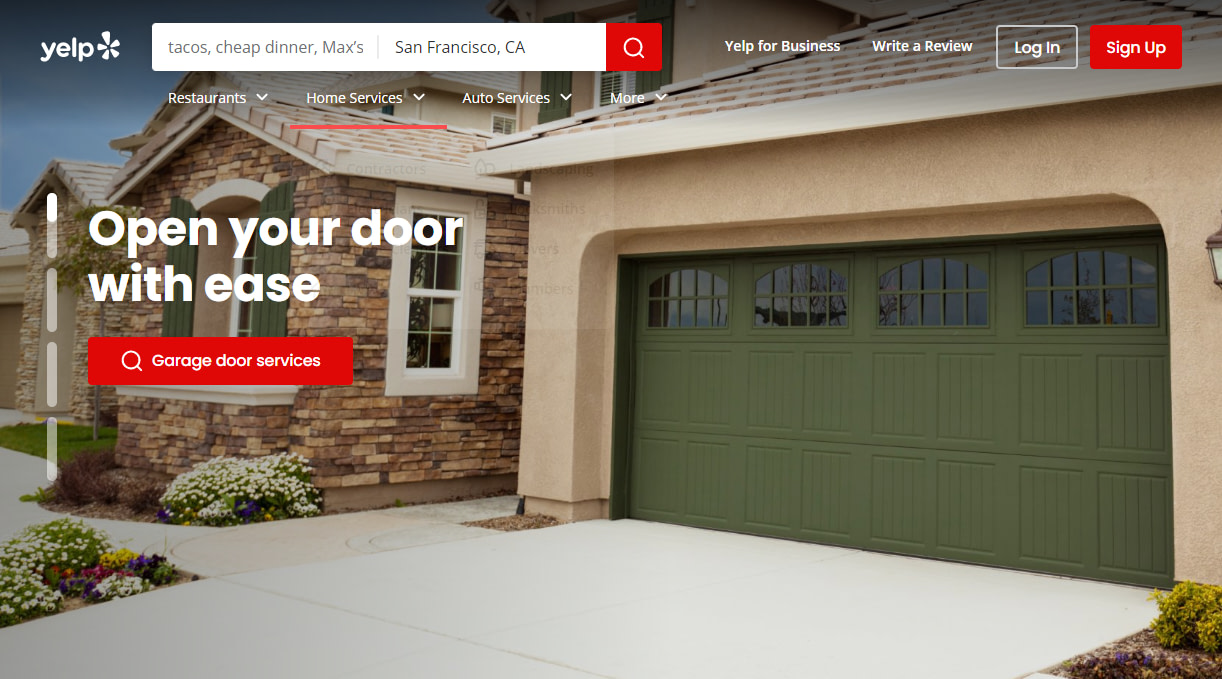This image is from the Yelp website, identifiable by the Yelp logo situated in the upper left corner. The search bar is populated with queries such as "tacos, cheap dinner, Max's, San Francisco, California." Prominent interface elements include tabs for "Write a Review" and "Yelp for Business," along with login and a conspicuous red and white sign-up button. There's a dropdown menu offering categories like "Restaurants," "Home Services," "Auto Services," and more.

The main section of the image features an advertisement banner with the text "Open Your Door with Ease." The banner includes a prominent red and white button labeled "Garage Door Services."

The background outdoor photo showcases a house constructed with dark and light brown bricks. In front of the house, a vibrant garden displays an array of flowers in white, blue, purple, yellow, red, and orange hues, complementing a patch of well-maintained grass. The house features a garage adorned with a green door, adding a splash of color to the overall scene.